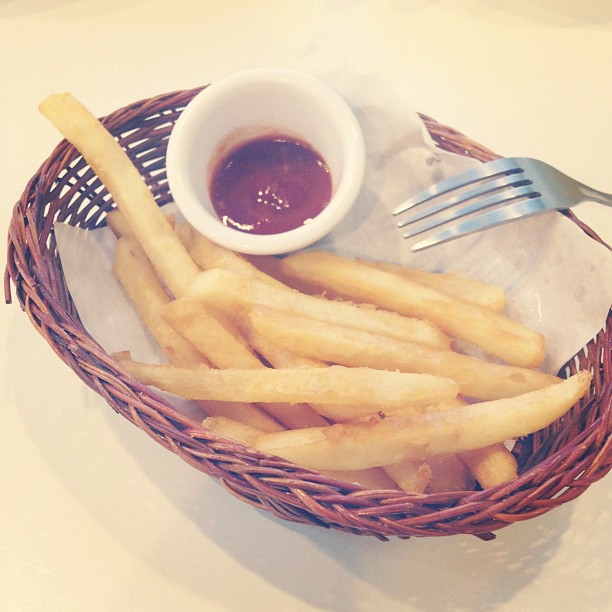In this faded, vintage-style photograph taken from above, a brown wicker basket holds a golden brown array of crispy French fries, lying atop a white liner. Tucked among the fries is a nearly-empty white ramekin of red ketchup. A silver fork extends from the right, hanging over the basket's edge, casting a shadow onto the bottom-right of the image. The basket's loosely woven structure allows glimpses of the background through its sides, emphasizing its rustic charm. The entire scene, with its muted colors and soft focus, exudes an old-fashioned, nostalgic aura.